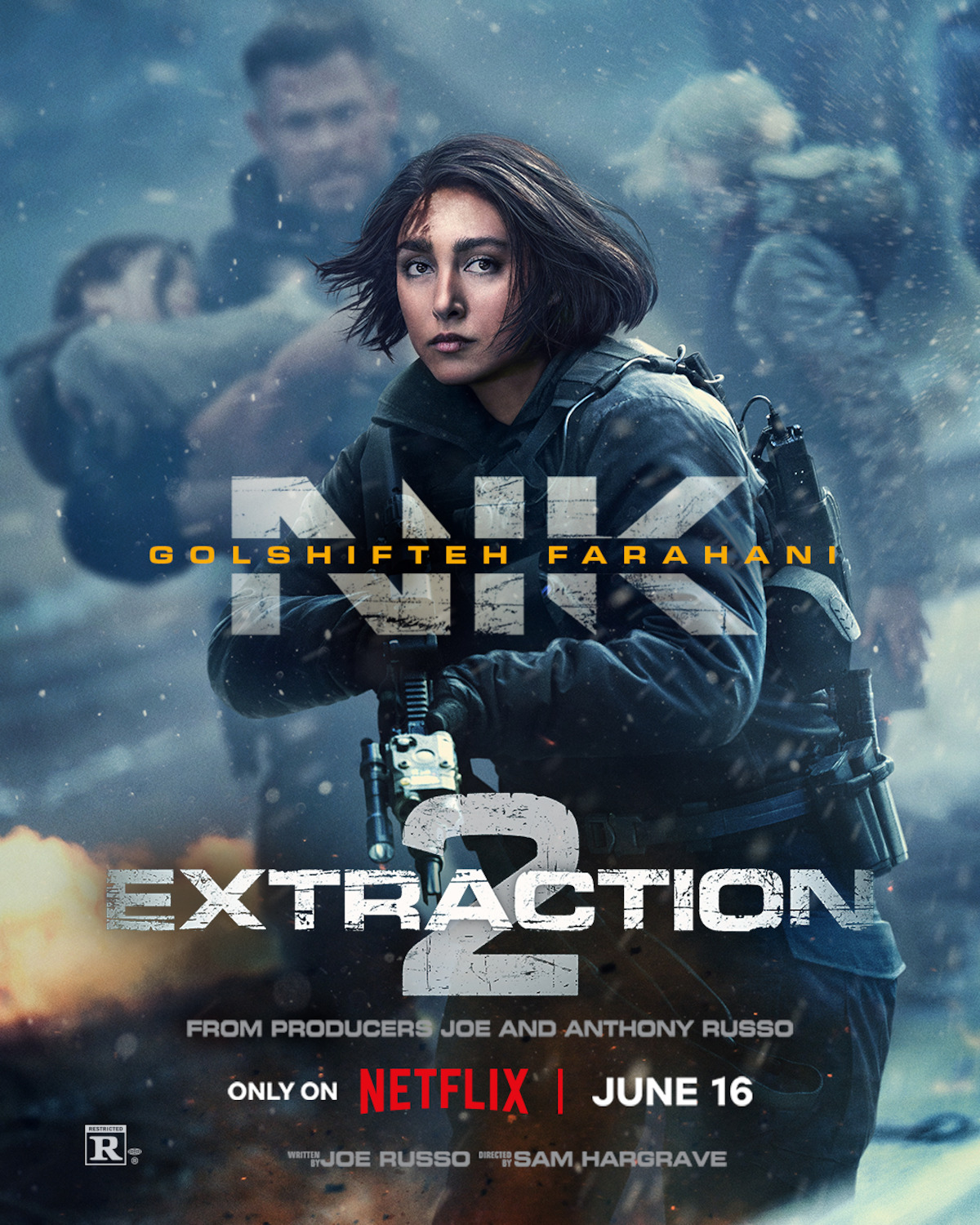The movie poster for "Extraction 2," premiering only on Netflix on June 16th, prominently features intense and dramatic imagery reflecting the high-stakes action of the film. The poster highlights a woman with short brown hair and blood on the left side of her forehead, dressed in tactical gear suitable for snowy conditions, holding a rifle with a determined stare. In the background, a man with short brown hair and facial hair, similarly dressed in tactical clothing, urgently carries a small child, emphasizing the perilous scenario. A blonde-haired woman, her hair blown by the wind, looks back anxiously at the chaos they're fleeing from, gripping a gun by her side. The setting suggests a combat zone amidst snow and an explosion of fire in the background, adding to the tension and urgency of their escape. The names of the producers, Joe and Anthony Russo, and the rating of R, are displayed, reinforcing the anticipation built around this upcoming release.